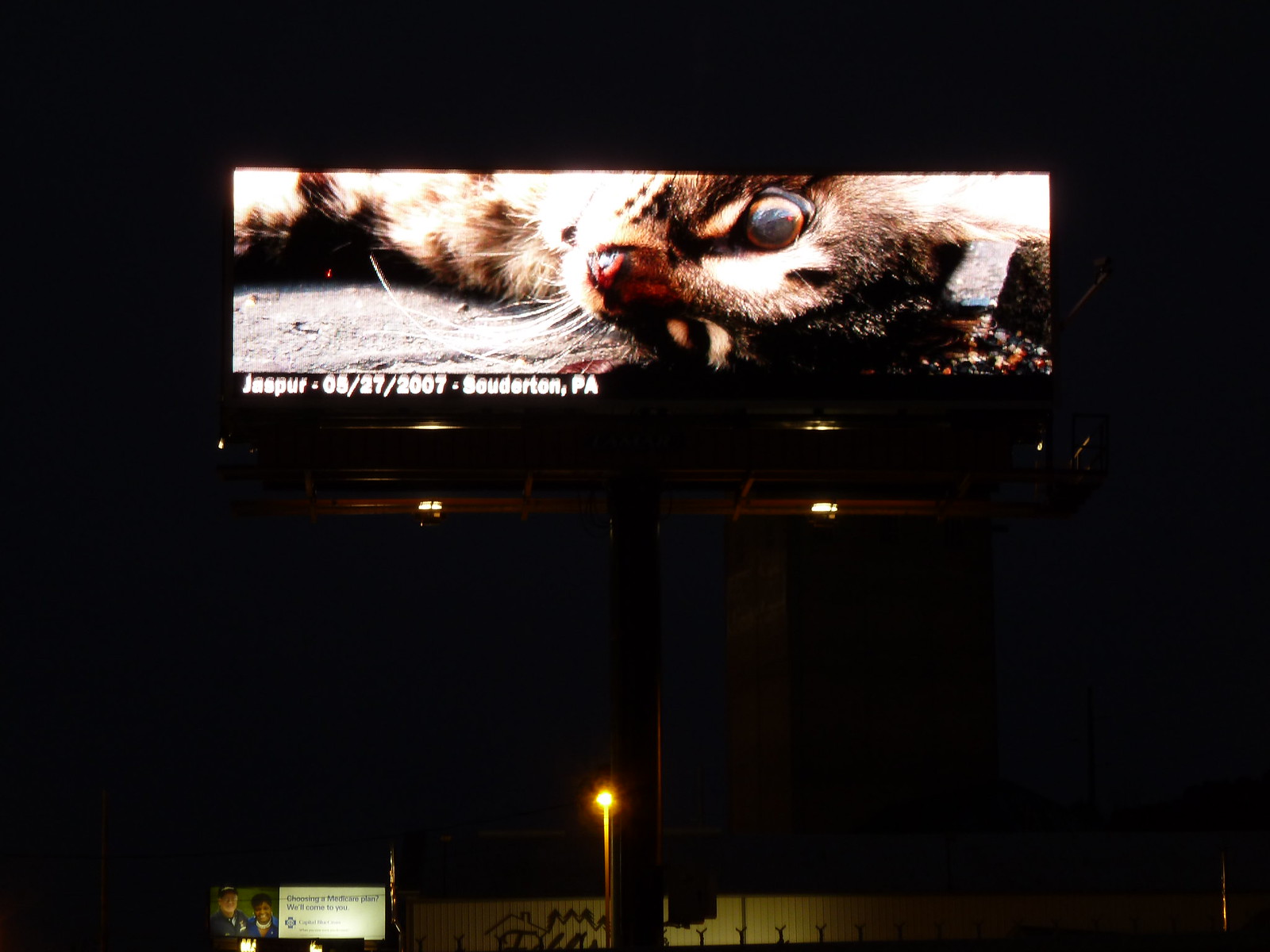The image captures a tall digital billboard mounted on a round metal pole with a solid metal base. The billboard is illuminated by two lights positioned on either side. The billboard's image depicts what appears to be an injured or deceased brown and white tabby cat lying on the ground. At the bottom left of the billboard, text reads "Jasper, 07-27-2007, Southerton, Pennsylvania." It's nighttime, and the setting is dark except for the illumination from the billboard itself. To the right in the background, a large building looms in the distance, while in the foreground, the top of a shorter building covered in graffiti is visible on the left. Additionally, a smaller, unreadable billboard can be seen in the lower left corner.